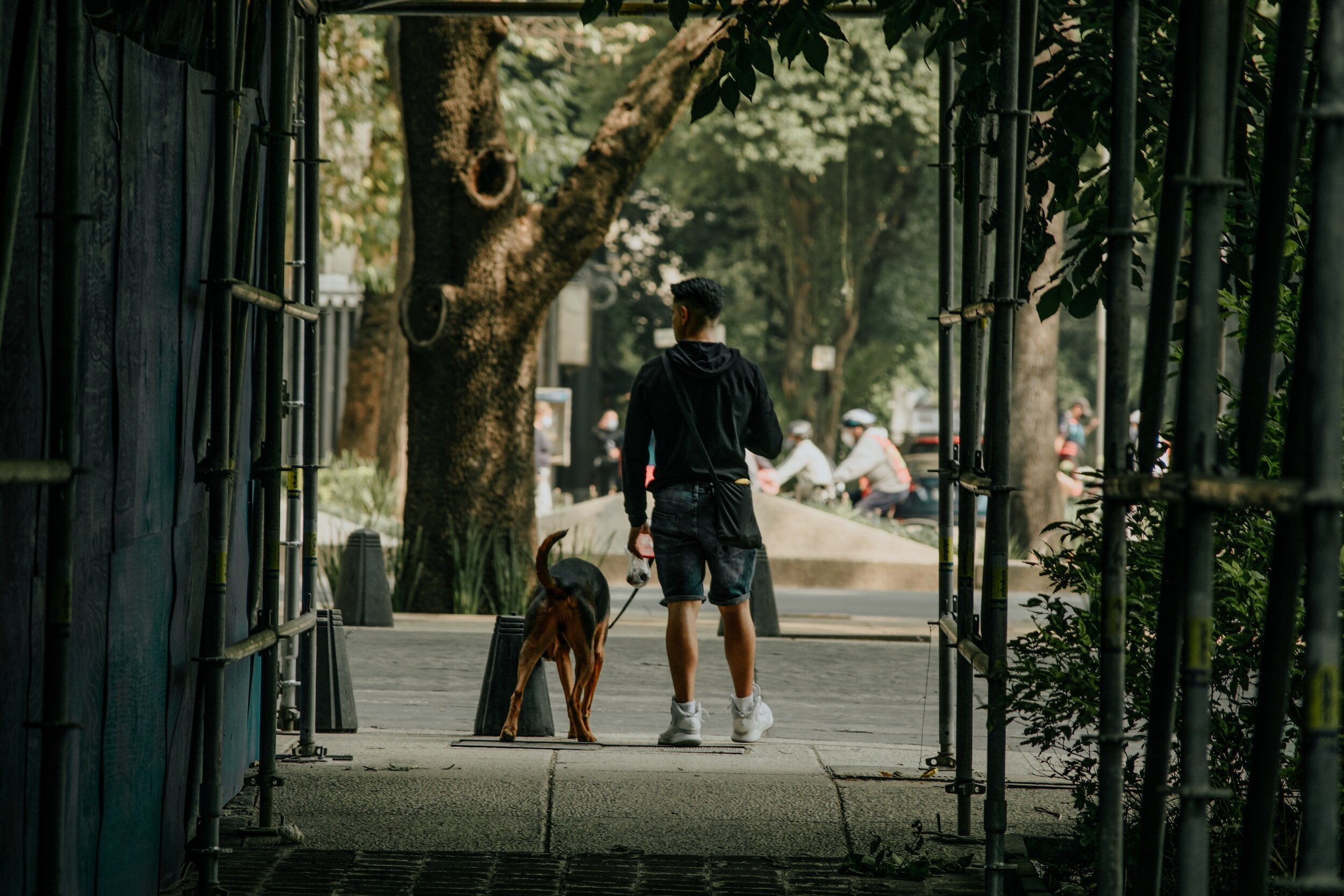This image captures a man walking a large, brown and black dog on a city sidewalk during the day. The focal point is the man, positioned toward the center of the image and facing away from the photographer. He is wearing a black sweatshirt, dark cargo shorts, and white high-top tennis shoes. In his right hand, he holds a leash attached to his dog, and possibly a cup of coffee or another item.

The setting is an urban environment, characterized by a street that they are about to cross and several elements that frame the scene. Across the street stands a large oak tree on a median, surrounded by other trees and greenery. In the background, blurred images of people, some on bicycles, and a few vehicles are observable. Further adding to the busy city atmosphere, a building with a partial fence is visible on the opposite side of the street.

The photograph appears to be taken from underneath a scaffold-like structure or a trellis adorned with metal gate doors and greenery, providing a natural frame for the shot. The overall weather condition seems warm and brightly lit, indicating daytime, without clear signs of direct sunlight.